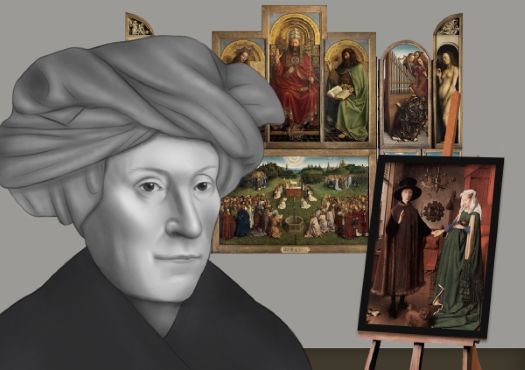The image depicts a 3D rendered scene featuring a central black and white figure, whose gender is ambiguous, with their head wrapped in what could be a towel, blanket, or turban. This figure occupies the middle left to bottom left of the frame, overlaying several framed paintings against a gray background. The figure’s position obscures some of these artworks. The paintings, which add vibrant colors to the scene including shades of green, red, beige, tan, and brown, depict various scenes: a couple holding hands, a religious figure, a group of people, a naked pregnant woman, someone playing a harp, and possibly others that are not entirely visible due to the central figure. The paintings are arranged in rows, some possibly resting on easels, and framed. The background includes a suggestion of texture or additional depth, contributing to the 3D effect. The overall setting combines a monochromatic primary figure with colorful, detailed paintings, creating a striking contrast.